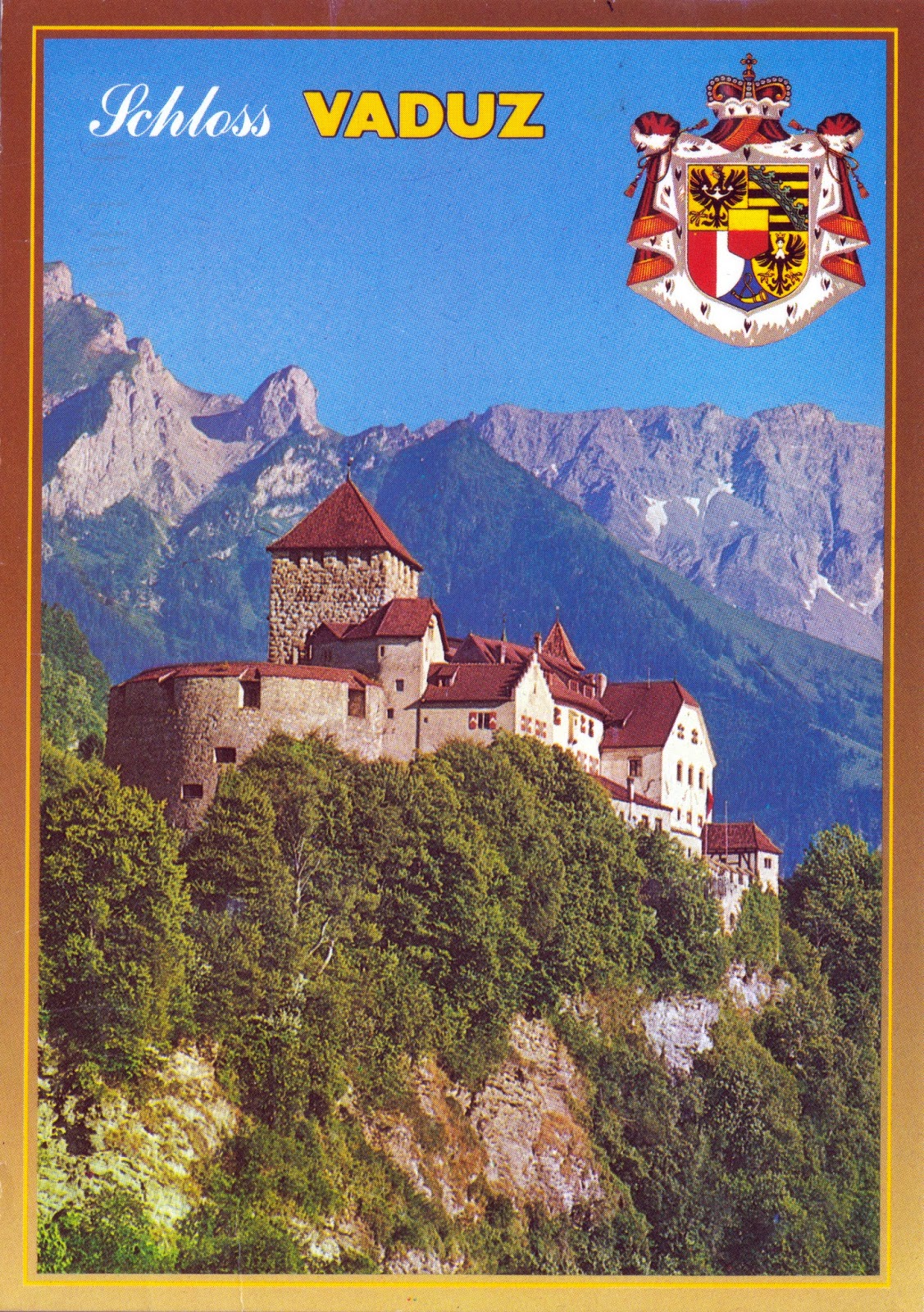This vertically oriented poster resembles a postcard and features a striking image of Schloss Vaduz, a majestic castle. The poster is framed with a gradient from brick-red at the top to yellow at the bottom, with a thin gold line running continuously around the photograph. At the top of the poster, "Schloss" is inscribed in cursive white script, followed by "VADUZ" in bold yellow uppercase letters on the right side. Adjacent to the text is a royal-looking crest adorned with a crown and draped fabric. 

The central photograph showcases the beige-stone castle with its red-brown roofs perched on a rugged cliff adorned with lush green trees. The castle itself features various architectural elements, including numerous windows, a circular section, and differing roof peaks. Beyond the castle, a breathtaking mountain range with a dusting of snow peaks into view, under a clear blue sky. The combination of the vividly colored frame and the detailed imagery creates a captivating and immersive visual experience.